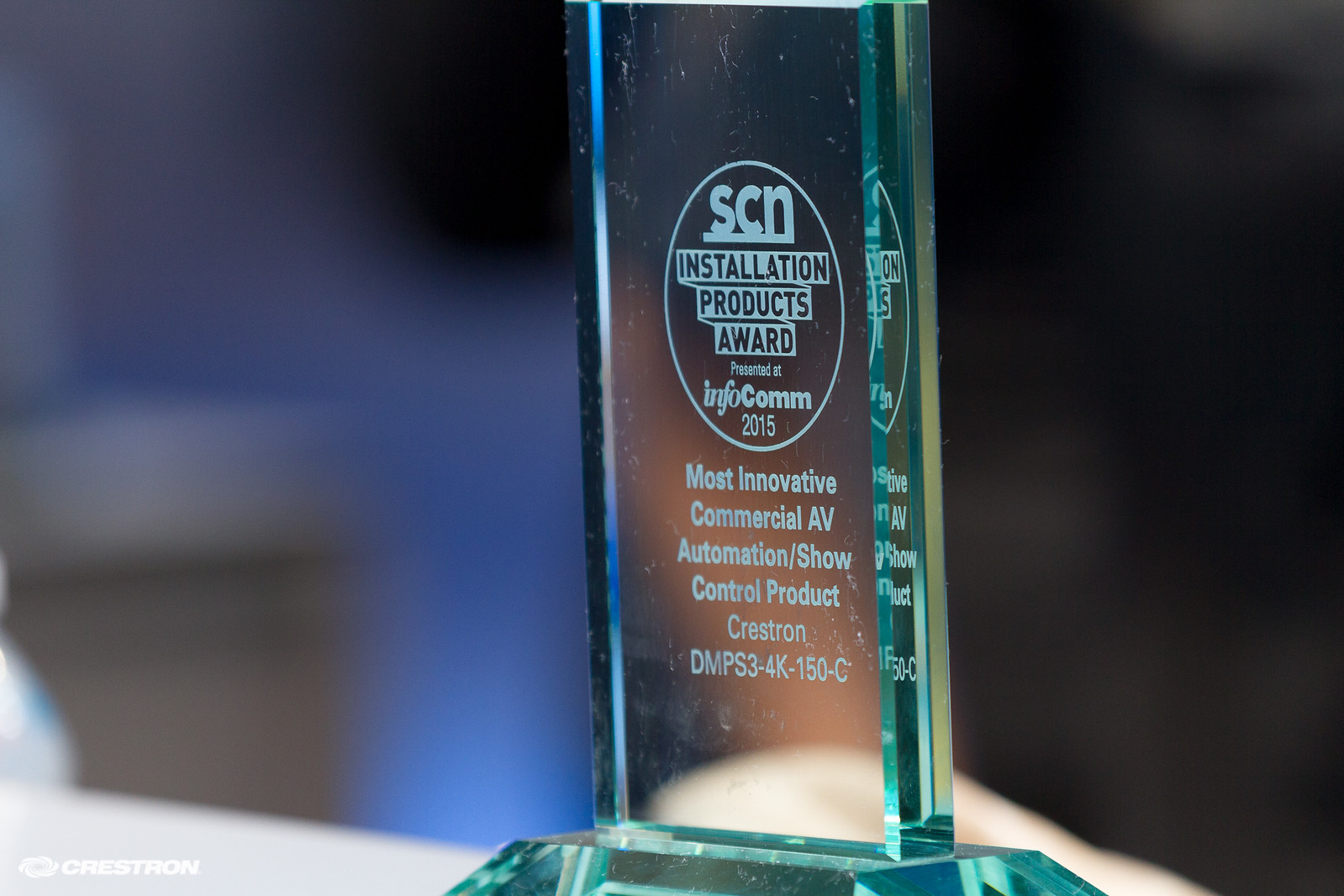The image is a close-up view of a clear glass award taken inside a room. The background is blurred, with blue hues on the left transitioning to darker shades on the right, and an indistinct counter or table on the left side. The award is prominently featured in the center, standing on a trapezoidal glass base and positioned on a white surface, which is partially visible in the bottom left corner along with a copyright or logo symbol that reads "Crestron."

Engraved in the middle of the glass award is a white circle containing various inscriptions. At the top, the underlined letters "SCN" are displayed, followed by "Installation Products Award" within a white banner, and "Infocomm 2015" beneath it. Further down, the text reads, "Most Innovative Commercial AV Automation/Show Control Product," followed by "Crestron DMPS3-4K-150-C." This detailed presentation indicates that the award was presented at the Infocomm 2015 event to recognize the most innovative commercial AV automation and show control product.